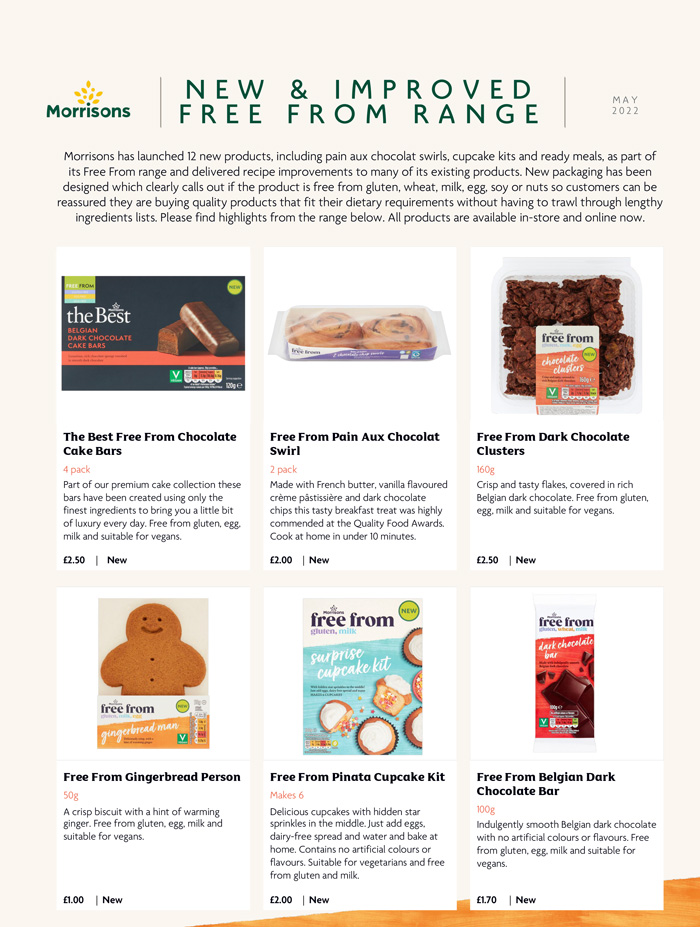This is an image showcasing Morrison's newly revamped 'Free From' product range as of May 2020. The top of the browser window indicates that Morrison's has launched 12 new items, including pain au chocolat swirls, chocolate swirls cupcake kits, and a variety of ready meals. This launch also involves significant recipe improvements to many existing products. 

The newly designed packaging prominently displays whether the product is free from gluten, wheat, milk, egg, soy, or nuts, making it easier for customers to identify suitable options without sifting through lengthy ingredient lists. Below the description, the layout features products arranged against a white background in a grid format, with three products per row over two rows. Featured items include:

- The best 'Free From' Chocolate Cake Bars (pack of 4)
- 'Free From' Pain au Chocolat Swirls
- 'Free From' Dark Chocolate Clusters
- 'Free From' Gingerbread Persons

All products from the 'Free From' range are available both in-store and online.